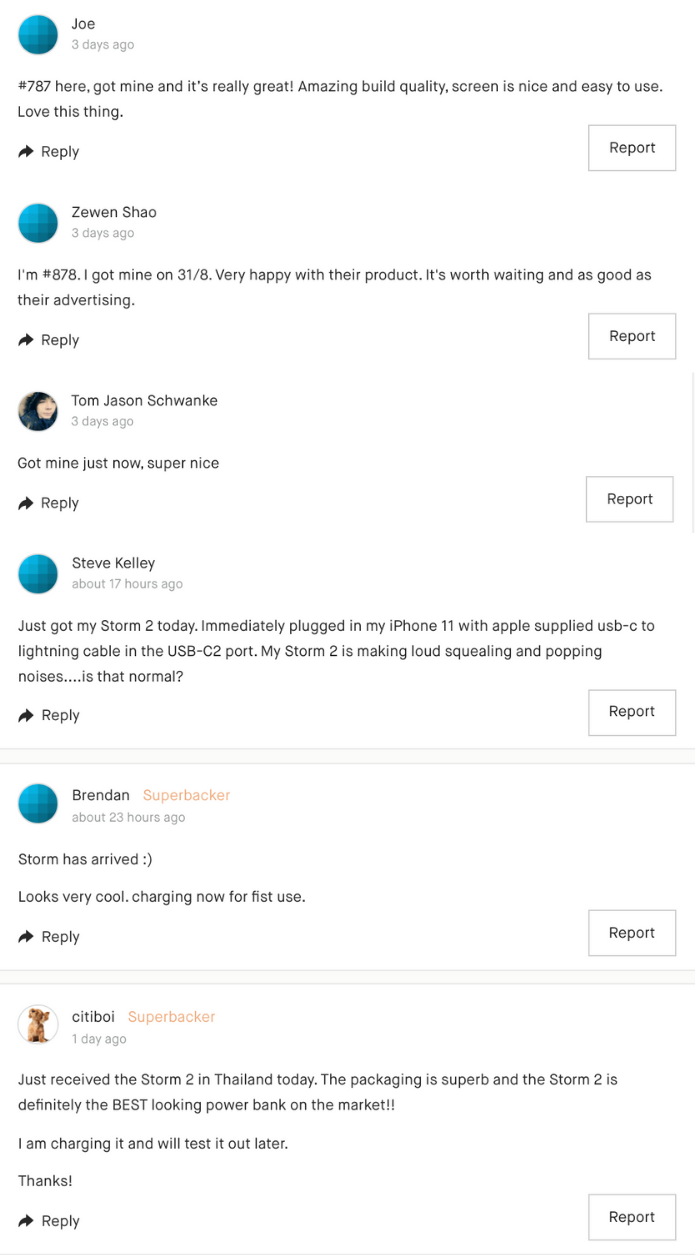This image depicts a lively conversation on a social networking or media platform, where multiple users are sharing their experiences with a newly released product, the Storm 2 power bank. At the top of the thread, user Joe, identified as Number 787, enthusiastically praises the device, noting its superb build quality and user-friendly screen. Below Joe's comment is user Ziwen Xiao, Number 878, who received their power bank on March 18th and is equally satisfied, affirming that the product lives up to the hype.

User Tom Jason Schwenke joins in to briefly confirm receipt of their unit, describing it as "super nice." However, the conversation takes a slight turn when user Steve Kelly reports an issue encountered with their Storm 2. Upon using an Apple-supplied USB-C to Lightning cable with an iPhone 11, they hear concerning squealing and popping noises from the device, prompting a query about whether this is normal behavior.

Amidst the technical concern, user Brendan shares their initial excitement, mentioning the arrival of their Storm 2 and their eagerness to begin its first charge, indicated by a smiley face. Lastly, user City Boy adds from Thailand, commending the exceptional packaging and aesthetic appeal of the Storm 2. They are currently charging the device and express anticipation for testing it out, ending their comment with gratitude.